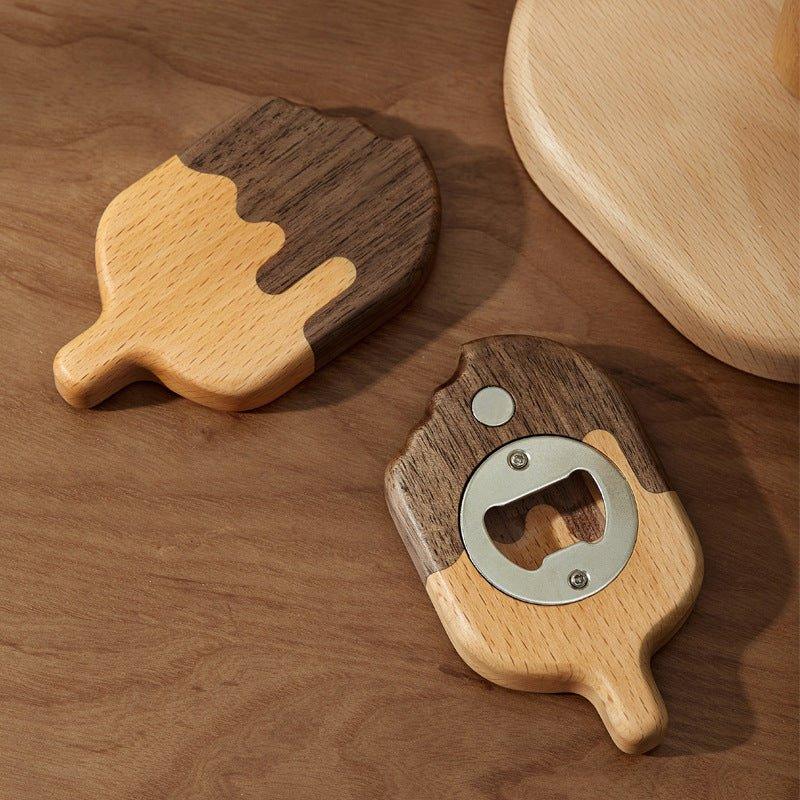This photograph features two intricately designed bottle openers shaped like ice cream bars, positioned on a medium brown wooden table. Both openers exhibit a creative design, making them resemble popsicles with a convincing twist. Each one has a polished wooden body divided into two sections: the top portion is a dark brown shade mimicking chocolate, artistically detailed to appear as if it’s dripping. The top left corner of the chocolate section even has a chunk missing, styled to simulate a bite mark. The lower section of these bottle openers is a natural light brown wooden stick. 

In the middle of one ice cream bar, a metallic silver bottle opener is embedded, marking it as the functional piece. The other ice cream-shaped object displays the same design but reveals the back, lacking the metal opener and instead presenting a smooth wooden surface. These pieces seem to serve not only as bottle openers but also as decorative magnets. 

To the right of these whimsical bottle openers, a lighter wooden surface—possibly a cutting board or tray—appears partially in the frame, though mostly cropped out. The entire setting rests atop a well-crafted wooden table, providing a warm and rustic background that complements the playful and artistic design of the bottle openers.